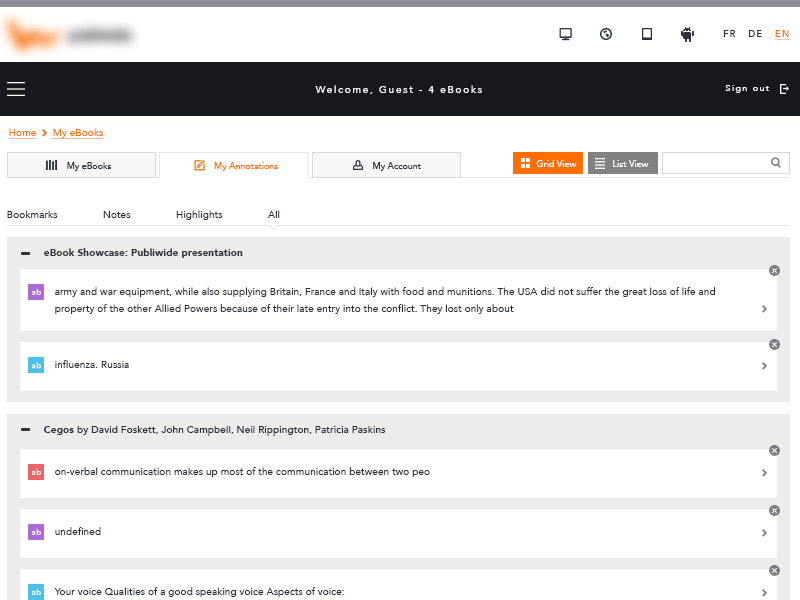The image features an interface related to e-books. The exact name of the site is obscured. At the top, the text reads, "Welcome Guest - 4 e-books," indicating that the user is logged in with an option to sign out. A language selection menu is present, with "EN" (English) highlighted in orange. 

Below this, there are several tabs: "My E-books," "My Annotations," "My Account," "Grid View," and "List View." The "My Annotations" tab is currently highlighted.

The main section of the interface displays a title, "E-books Showcase: Public Wide Presentation," followed by a list of e-books. The first e-book is titled, "Army and War Equipment: Supplying Britain, France, and Italy with Food and Munitions," with a brief description that the USA did not experience the same level of loss in life and property as other Allied Powers due to its late entry into the conflict, ending mid-sentence.

Below that, the titles "Influenza, Russia" and "Seagulls by David Foskett, John Campbell, Neil Reppenton, and Patricia Raskins" are listed, the latter with three associated sections.